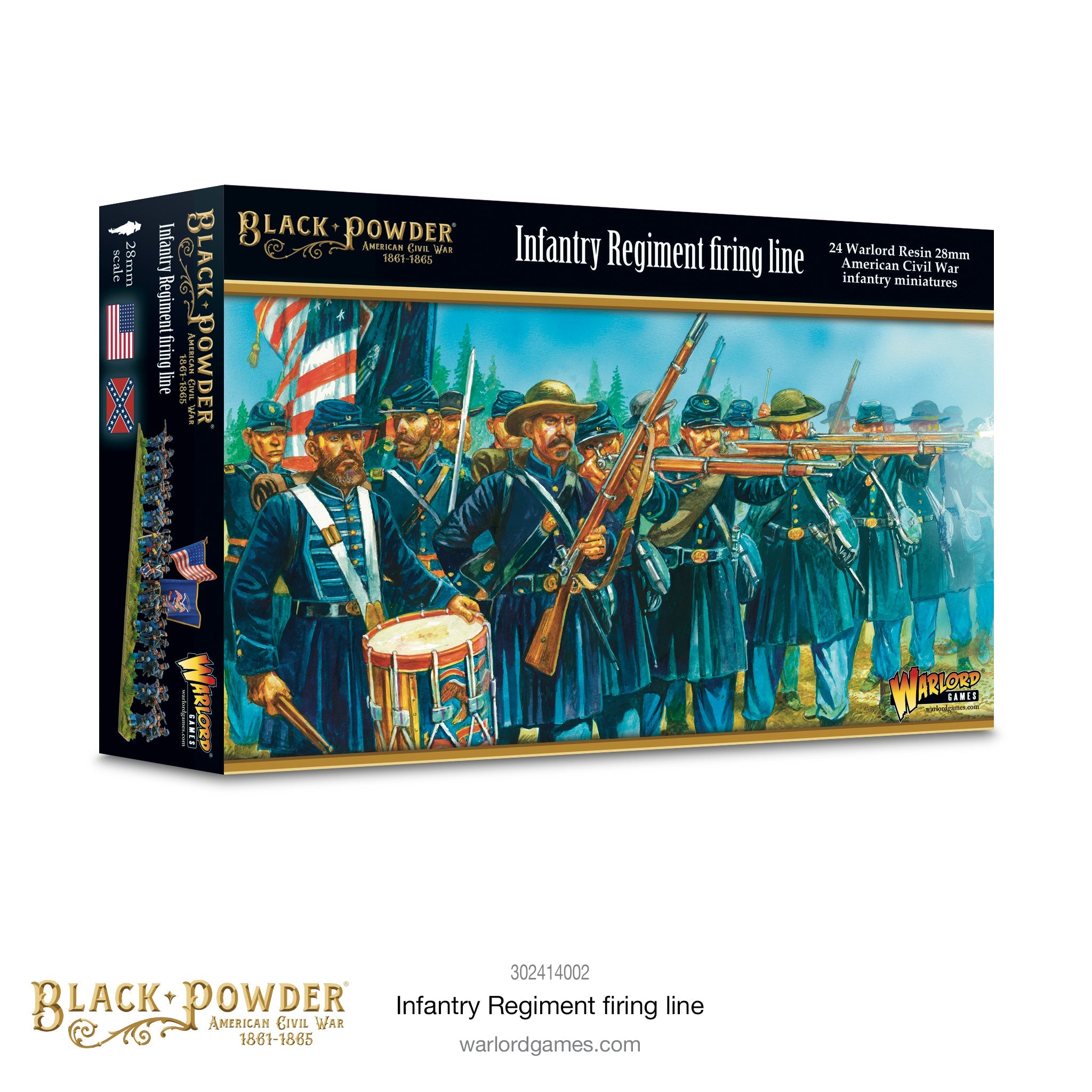The image depicts a rectangular box with a detailed illustration related to the American Civil War. The box, which houses 24 American Civil War infantry miniatures, prominently features soldiers in blue Union uniforms, with some depicted firing or reloading their rifles, and one soldier holding a drum. The figures are part of a "Black Powder" series by Warlord Games. 

The box's front cover is dominated by a scene of soldiers on a firing line, with a black background at the top and a gold bar underneath. Inscribed in gold text is "Black Powder American Civil War 1861-1865," and below it in white text, "Infantry Regiment Firing Line." The top right corner includes the specifics: "24 Warlord Resin 28mm American Civil War Infantry Miniatures." The side of the box mirrors this information and features both an American and a Confederate flag.

Additional labels include "Warlord Games" in the lower right corner and product number "302414002" with the website "WarlordGames.com" on the lower front side. The uniform details reveal variations, with some soldiers wearing tan hats and others blue caps.